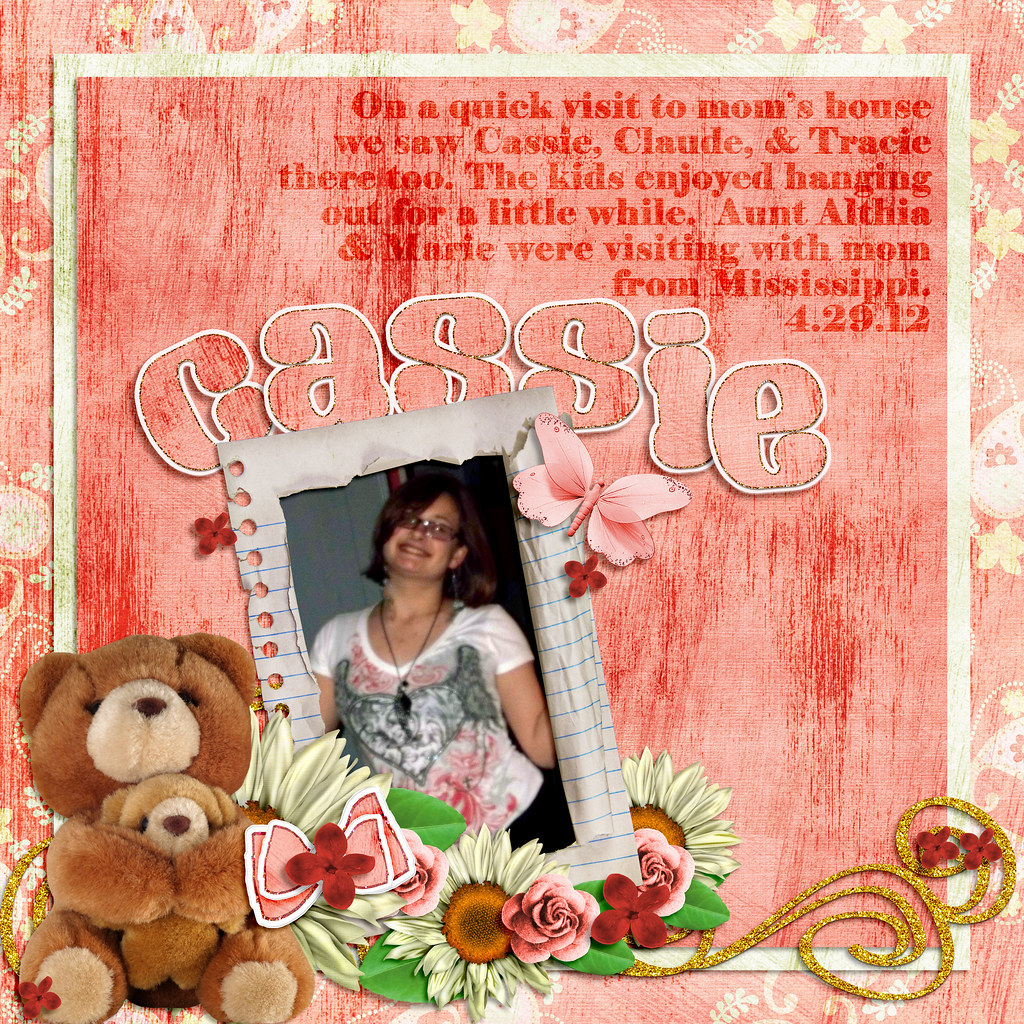This square digital scrapbook card features a light pinkish-red background adorned with a delicate pattern of pastel yellow flowers, complete with tiny leaves and whimsical strings. Central to the design is a light yellow frame housing a pinkish-yellow pattern embossed with large, bubble letters reading "Cassie," surrounded by a crisp white outline. In front of this name is a picture of a girl with short brown hair and glasses, wearing a white shirt with a gray and pink design topped off with a necklace. She's smiling and has her head tilted slightly, and the photo appears to be torn and pasted onto a torn notebook page, adding a nostalgic touch.

Bordering the flower-filled background are images of teddy bears and blossoms. The scrapbook card's top right corner contains red text: "On a quick visit to mom's house we saw Cassie, Claude, and Tracy there too. The kids enjoyed hanging out for a little while. Aunt Althea and Mary were visiting with mom from Mississippi." This vibrant, intricate card captures a precious memory and radiates warmth and family togetherness.